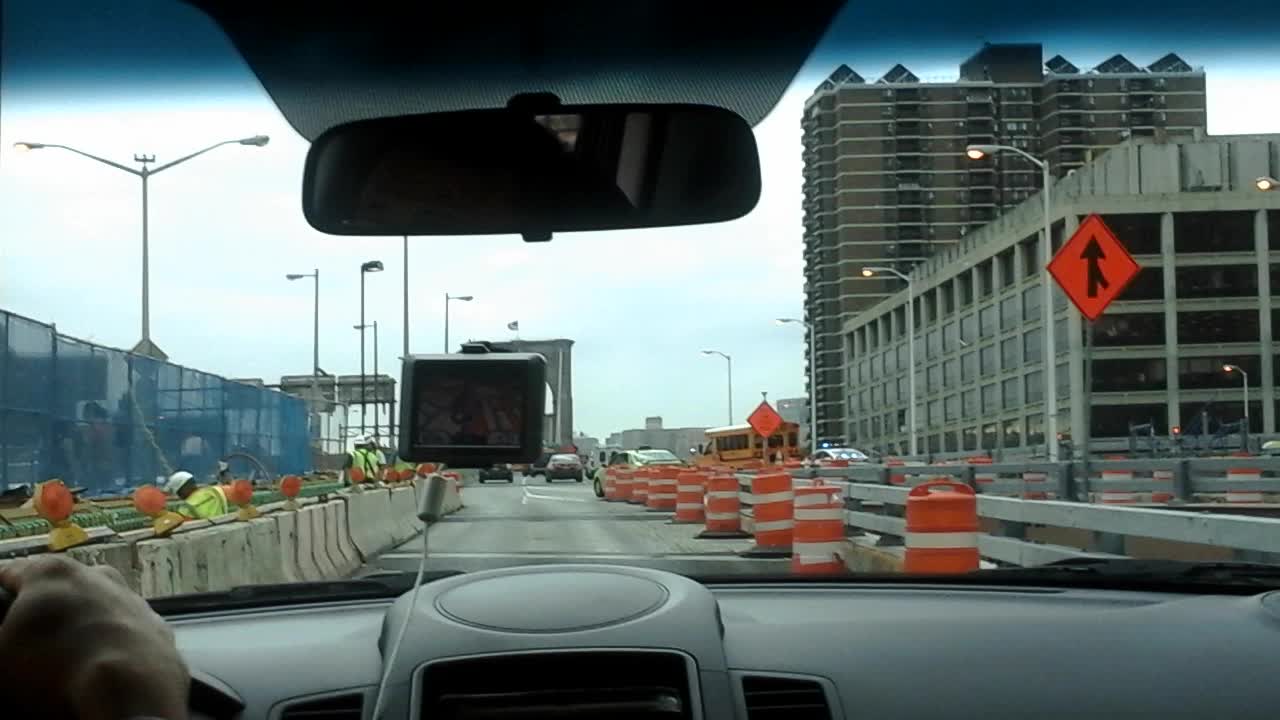The image is a photograph captured from the interior of a car, likely from the midpoint, offering a centered view through the front windshield. Inside the vehicle, the gray dashboard stretches out in front, while at the top of the frame, the rearview mirror hangs, reflecting mostly indistinguishable dark shapes. Below the mirror, a GPS unit is affixed to the windshield via a suction cup, with a white cord dangling from it. A fair-skinned hand, presumably the driver's right hand, rests on the visible steering wheel to the left.

Outside the car, a city street stretches ahead, currently under construction. On the right side of the road are numerous orange and white traffic barrels. To the left, a line of concrete jersey barriers separates the road from a group of construction workers. The workers are easily identifiable in their high-visibility yellow shirts and white hard hats. Behind the barriers, partial views of tall buildings—possibly a high-rise office building or apartment complex—and a multi-level parking garage dominate the skyline. Streetlights and additional fencing are also visible along the construction area, adding to the urban scene.